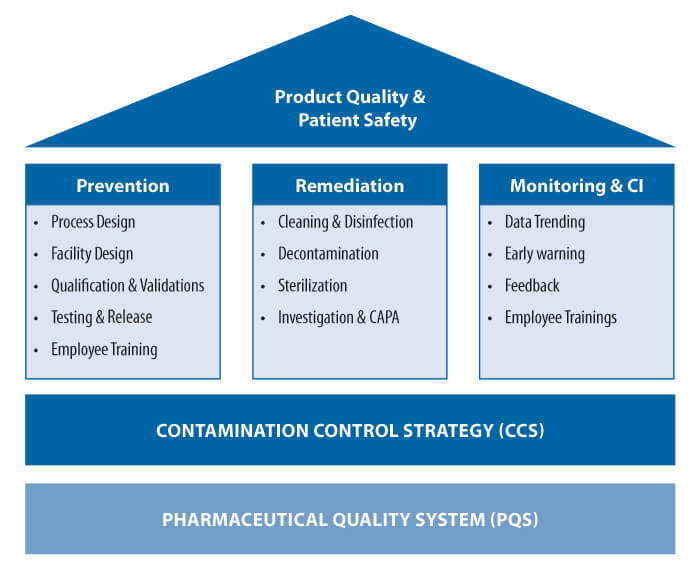The infographic prominently titled "Product Quality and Patient Safety" is detailed in various shades of blue, featuring multiple geometric shapes. At the top center, a blue triangle highlights the main theme. Below it, three dark blue rectangles are displayed side by side. The first rectangle, labeled "Prevention," contains sections for Process Design, Facility Design, Qualifications and Validations, Testing and Release, and Employee Training. The middle rectangle, labeled "Remediation," includes Cleaning and Disinfection, Decontamination, Sterilization, Investigation and CAPA. The third rectangle, labeled "Monitoring and CI," lists Data Trending, Early Warning, Feedback, and Employee Training. Beneath these, two larger rectangles appear: one dark blue rectangle labeled "Contamination Control Strategy (CCS)" and, at the bottom, a lighter blue rectangle labeled "Pharmaceutical Quality System (PQS)." The entire design is cohesive, emphasizing key processes for maintaining high standards in product quality and patient safety.